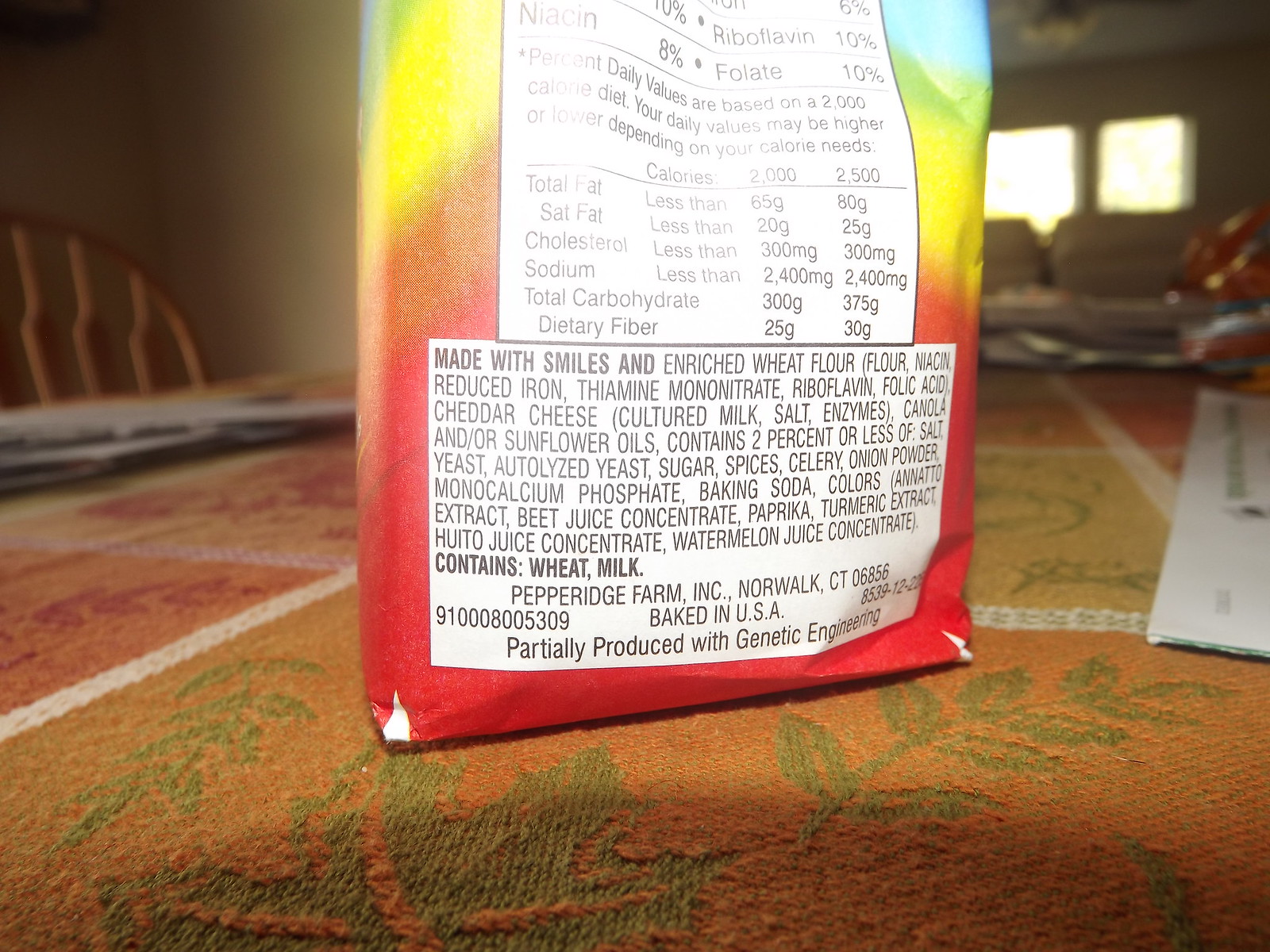The image captures a Pepperidge Farm snack product prominently placed on a dining table in a home setting. The table is adorned with a festive fall-themed tablecloth featuring a vibrant mix of orange, yellow, red, and green leaves. There are a few miscellaneous items, such as envelopes, scattered on the table. A wooden dining chair is partially visible, positioned next to the table. In the background, a couch can be seen, contributing to the cozy, lived-in atmosphere of the scene.

The Pepperidge Farm product appears to be some kind of cheddar cheese-flavored cracker snack, likely intended for children, based on the ingredients list which includes cheddar cheese, milk, and flour. The packaging displays nutritional facts, albeit some parts are slightly obscured. Notably, the product is labeled as "Baked in the USA."